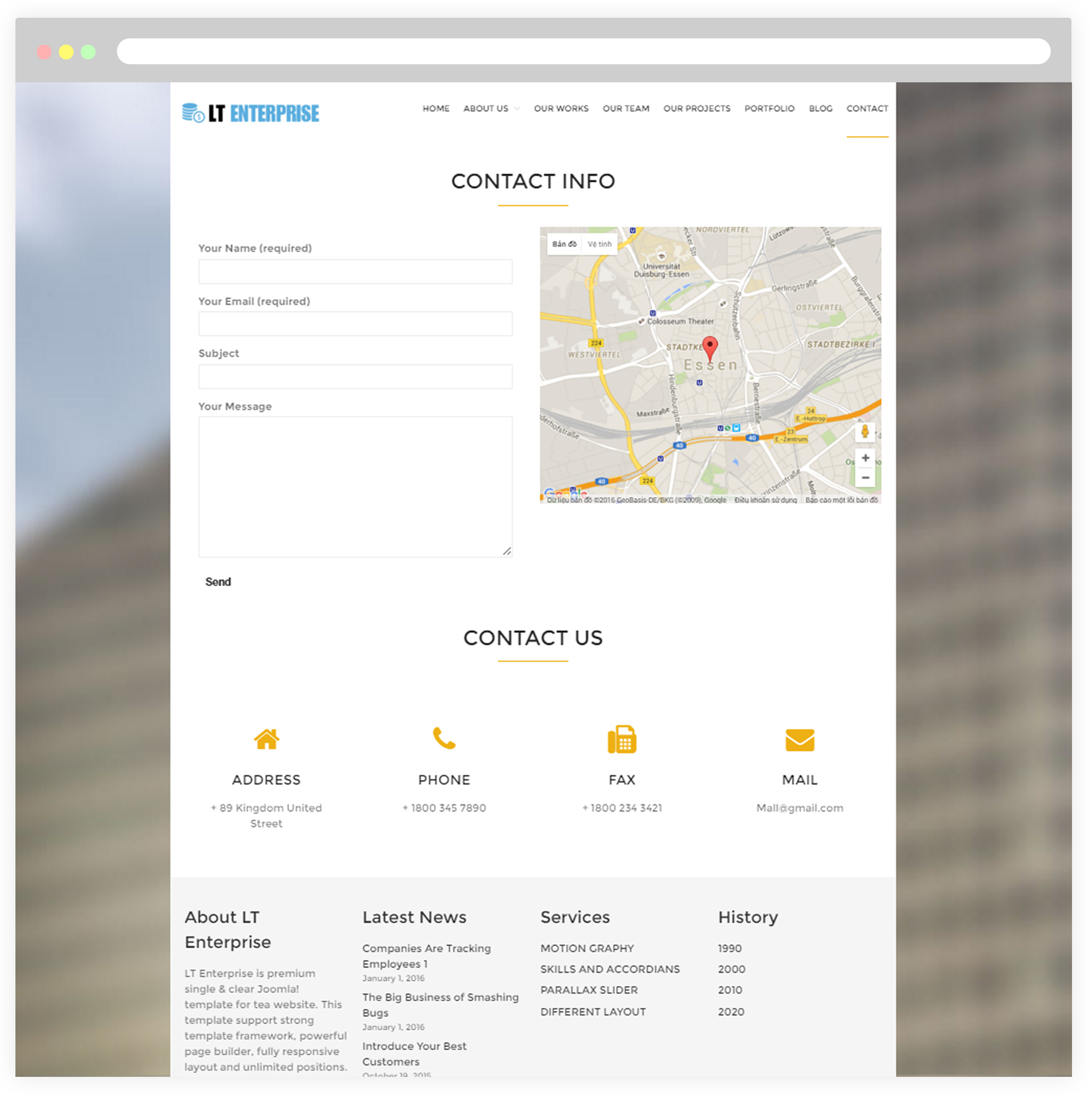This is a detailed screenshot of a Safari browser window showcasing the contact page of the LT Enterprise website. 

At the very top, the browser’s address bar is visible. The page’s content features a background image, mostly obscured by a white overlay box. Inside this white box, the LT Enterprise logo appears at the top left corner, featuring "LT" in black and "Enterprise" in blue, accompanied by a stack of coins symbolizing the brand logo.

A menu bar is situated to the right of the logo, containing navigation options: Home, About Us, Our Works, Our Team, Our Projects, Portfolio, Blog, and Contact. The "Contact" menu option is underlined in yellow, indicating the active page. Below the menu bar, "Contact Info" is prominently displayed in uppercase black text, emphasized by a small yellow underline.

On the right side of the page, there are input fields for "Your Name," "Your Email," "Subject," and "Your Message," intended for visitor queries or messages. Adjacent to these text boxes is an embedded map centered on Essen, marked by a pinpoint location indicator.

Underneath the initial content, the "Contact Us" section features a row of icons providing relevant contact information from left to right: an address icon followed by "89 Kingdom United Street," a phone icon with the number "1-800-345-7890," a fax icon with "1-800-234-3421," and a mail icon with the email address "mail@gmail.com."

At the bottom of the page is the footer, divided into four columns:
1. **About LT Enterprise**: Contains information about the company.
2. **Latest News**: Lists three articles, all dated January 1, 2016.
3. **Services**: Indicates four service offerings, including "Motion Graphing."
4. **History**: Lists significant dates from 1990 to 2020. 

Overall, the screenshot captures a highly organized and detailed contact page designed for ease of navigation and user interaction.